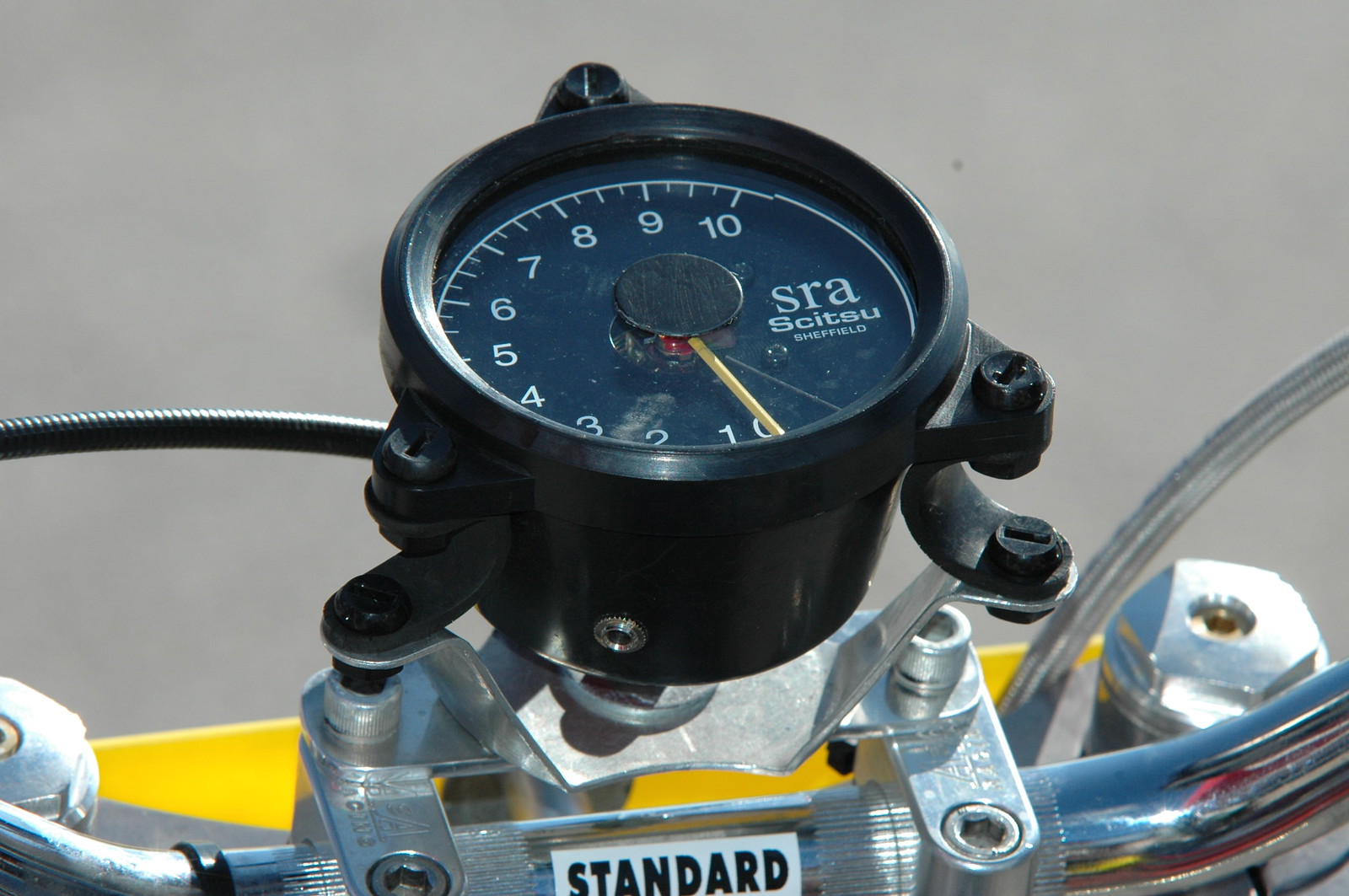This image features a detailed close-up of a gauge set against a white background. Dominating the foreground is a black dial with white numerals ranging from 1 to 10, possibly indicating pressure levels. The gauge includes a yellow needle pointing to a specific value. The face of the gauge is black, with the white text "SRA" prominently displayed, followed by "SKITZU" in a smaller font and "SHEFFIELD" in very small letters below, suggesting the place of manufacture.

To the left side of the gauge, there is a thin metal component, while a silver metal piece is partially visible on the right side of the image, mostly cut off from view. Towards the bottom of the gauge, the word "STANDARD" is clearly printed in a bold black font against a white background. The overall setting appears to be either outdoors or within a well-lit building.